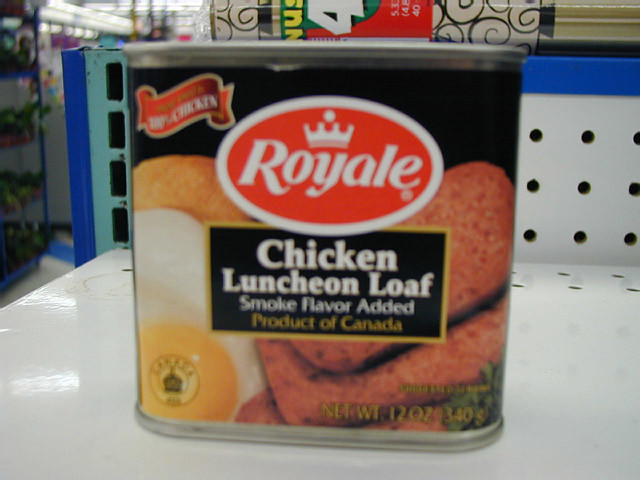A tin can of Royale Chicken Luncheon Loaf is neatly placed on the top shelf of a grocery store. The shelf features a white surface with a perforated back wall. The can's label prominently displays an appetizing image of the luncheon loaf, with three slices arranged next to fried eggs. The Royale brand logo, an oval red circle outlined in white, is positioned in the center, with the brand name “Royale” written in white letters and topped by a crown with a dot. In the bottom right corner of the label, the net weight is indicated in yellow print, stating "12 ounces (340 grams)." Additionally, a round logo featuring "Canada" is found on the bottom left side of the can.